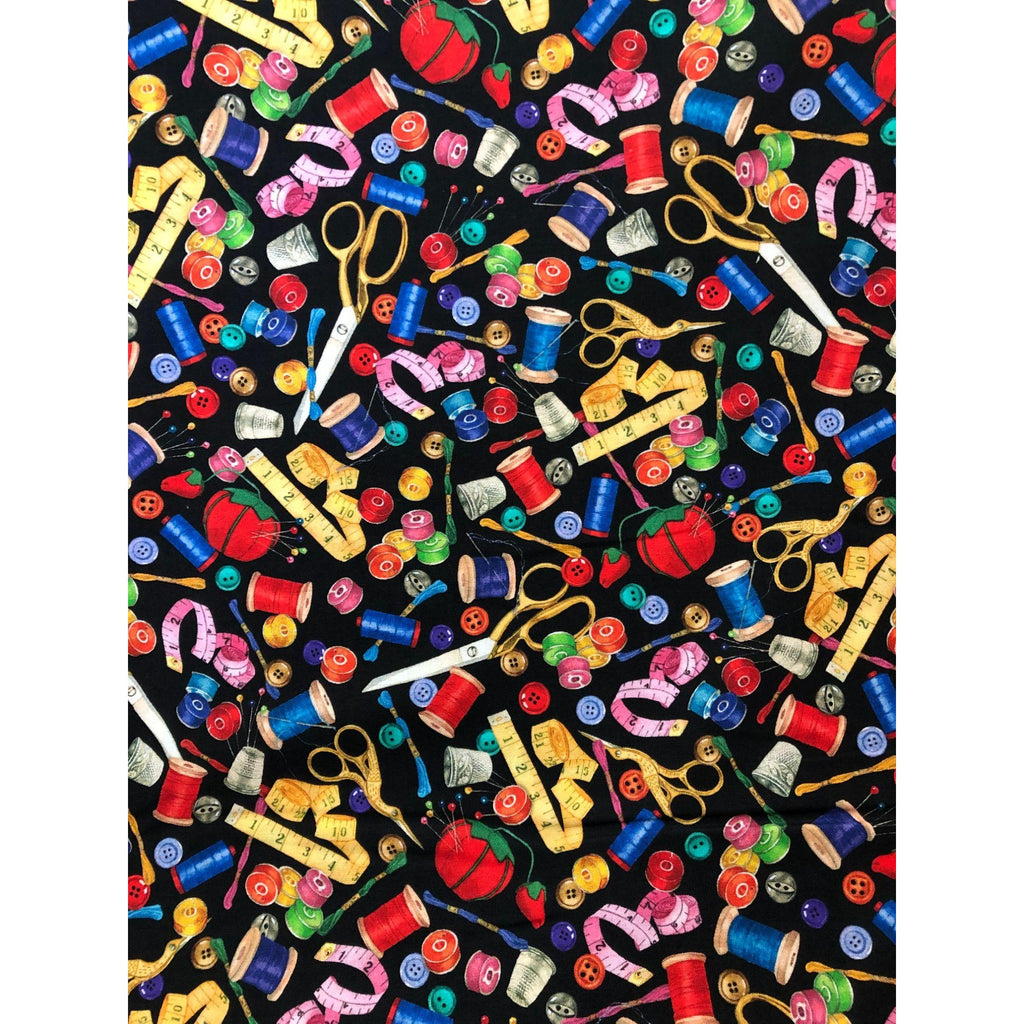The image captures an overhead view of a black background densely scattered with various colorful sewing notions, creating a vibrant and repetitive pattern. Prominent among these are gold-handled scissors with silver tips, including some uniquely curved pairs. There are also multiple tape measures in yellow and pink, spools of thread in shades of dark blue, light blue, red, green, and orange, and a myriad of buttons in assorted colors. Adding to the array are bobbins holding red, yellow, and green threads, and classic tomato-shaped pin cushions punctuated with silver pins. These sewing materials are meticulously arranged in a repetitive, kaleidoscopic manner, forming a lively tapestry of rainbow hues against the stark black backdrop.